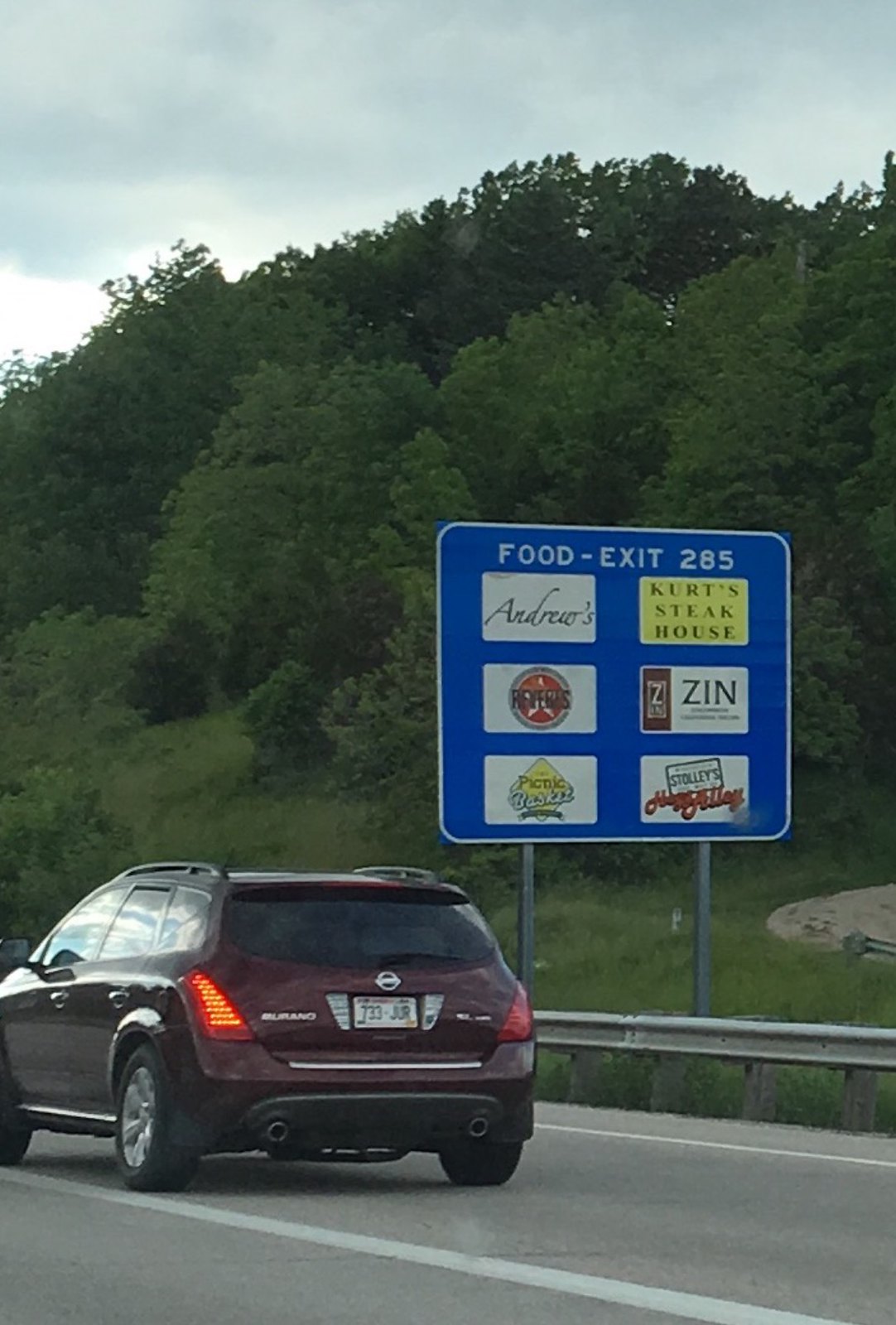A detailed road sign stands prominently against a backdrop of lush, green trees and rolling hills, as seen from the driver's or passenger's side of a car traveling on a highway. In the foreground, a red or dark red hatchback—a four-door vehicle lower than a minivan—signals a left turn, continuing along the same route.

The blue road sign, indicating "Food and Exit 285," showcases six different food options available at that exit:

1. **Andrews:** A white sign with elegant green cursive writing.
2. **Kurt's Steakhouse:** A distinctive yellow sign with bold green lettering.
3. **Reveres:** A circular sign characterized by a red interior and a central white star.
4. **Zin:** A vertically oriented brown rectangle, featuring a large "Z" at the top and "Zin" underneath, accompanied by additional smaller text that is not fully visible.
5. **Picnic Basket:** A creatively designed white sign with a yellow diamond, featuring the word "Picnic" in dark blue print and "Basket" in white cursive outlined in blue.
6. **Stolley's:** A sign with the inscription "Stolley's" in prominent letters followed by "License Plate" and partially visible text indicating "Something Alley."

This captivating image captures the attention with its layered details, combining natural beauty with practical road trip information.